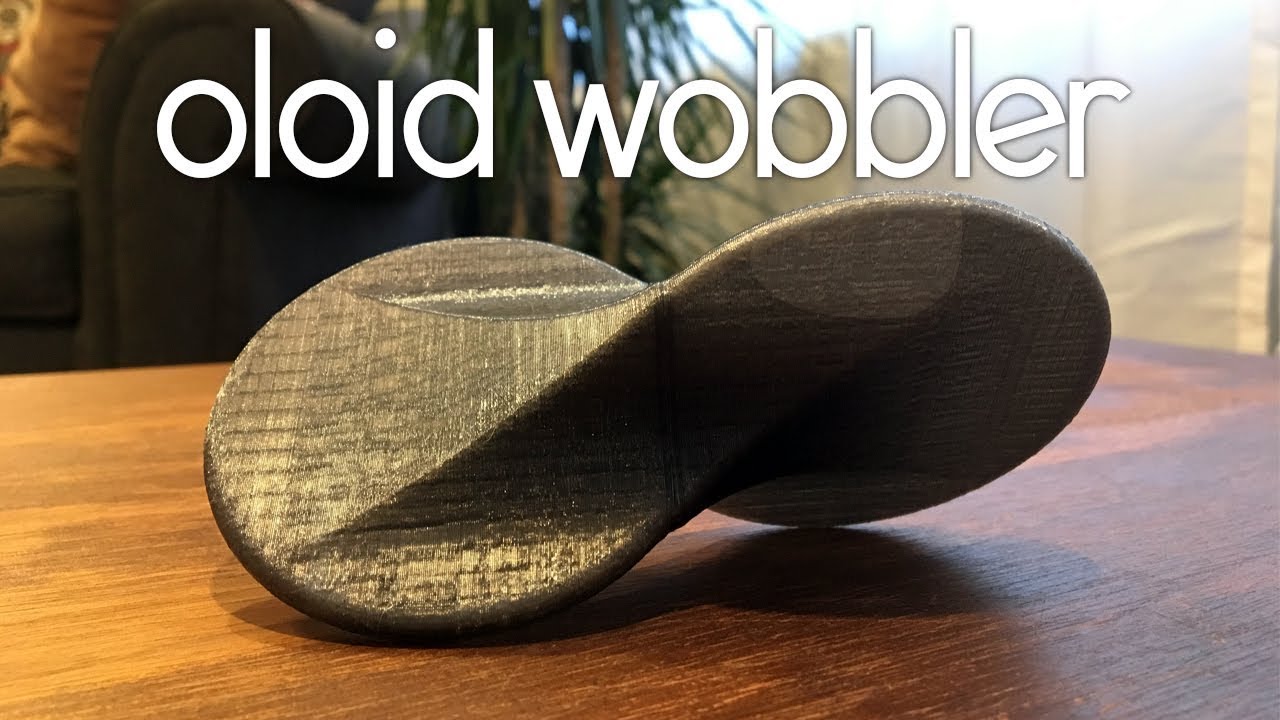This indoor photograph, rectangular in shape (approximately six inches wide and three inches high), features a light brown wooden table occupying the lower half of the image. The left side of the table showcases a golden brown hue transitioning to a deeper, flat brown as it progresses to the right. Centered on this table is a unique statue, potentially crafted from stone or metal, shaped like an elongated figure-eight with a quarter-turn twist. The statue's left side, covered in a shiny, metallic gray, contrasts with its shadowed right side. In the background, to the left, part of a chair is visible, while the center is dominated by a houseplant. The right side fades into a blur influenced by sunlight streaming in, coupled with the bright sky outside. Bold white text across the top reads "Oloid Wobbler," with "Oloid" spelled O-L-O-I-D.